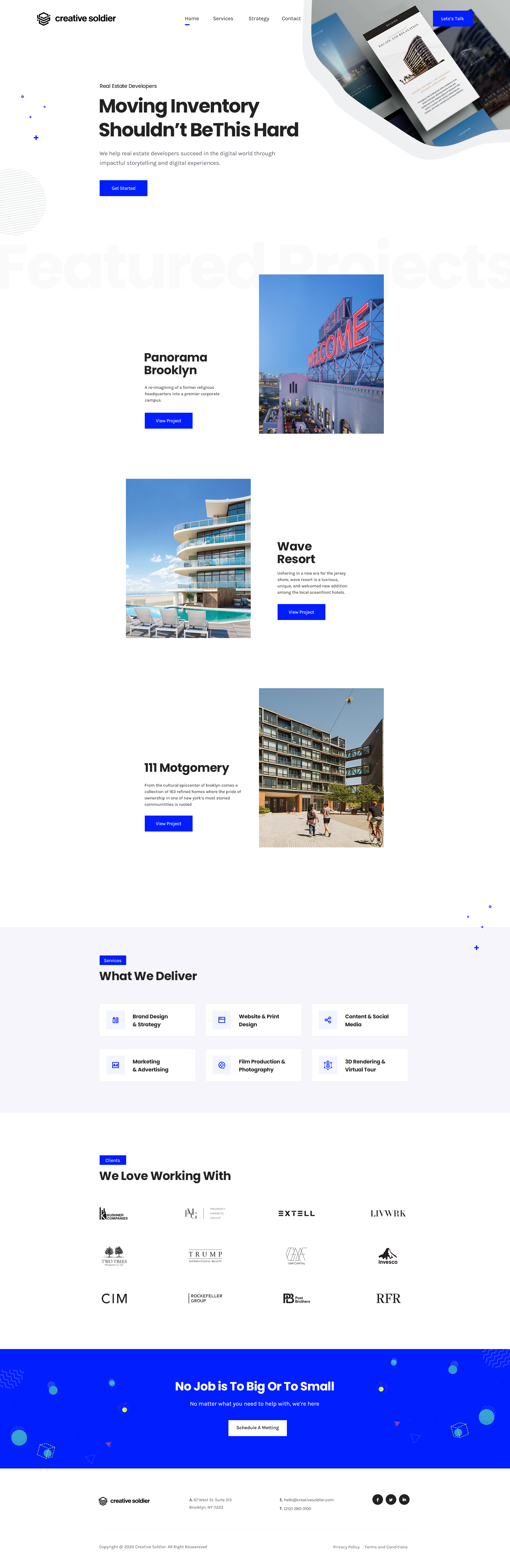"Creative Soldier Website Overview"

The Creative Soldier website, evocatively branded with an army theme, features a sleek and modern design. The main navigation bar, located at the top right, includes buttons for Home, Service, Strategy, and Contact. Currently, the 'Home' section is active, indicated by a subtle blue underline beneath it.

To the right of the 'Contact' button, in the upper right corner of the page, there is a large, diagonally-arranged, slightly triangular section. This features an image showcasing various smartphone snippets. The section is titled "Escape and Relaxation" and displays an impressive tall condominium with a brief, unreadable description. Adjacent to this is a call-to-action labeled "Let's Talk" with a prominent blue button.

Further down to the left, the phrase "Real estate developers rule small" faintly appears, followed by a bold statement, "Moving inventory shouldn't be this hard." This headline is split over two lines, emphasizing the difficulties in inventory movement. Below this, a succinct mission statement reads: "We help real estate developers succeed in the digital world through impactful storytelling and digital experiences," accompanied by another blue call-to-action button, "Get Started."

An image of a large digital sign that says "Welcome" is positioned next to a group of people walking around a building’s perimeter patio. Left of this image, text reads "Panorama Brooklyn, reimagined from a former religious headquarters," alongside a "View Project" link. Featured projects also include "Wave Resort," complete with an image and "View Project" link, and "111 Montgomery" with an image but no further link.

A comprehensive box below lists the services provided by Creative Soldier: Brand Design and Strategy, Marketing and Advertisement, Website and Print, Film Production, Content and Social Media, and 3D Rendering. The "Clients" section follows, showcasing the diverse range of clients they have worked with. At the bottom, a vibrant blue box declares, "No job is too big or small," accompanied by a "Schedule a Meeting" prompt within a white-bordered button. The page concludes with the company's contact information, including a phone number and address, ensuring all pertinent details about the business are readily accessible.